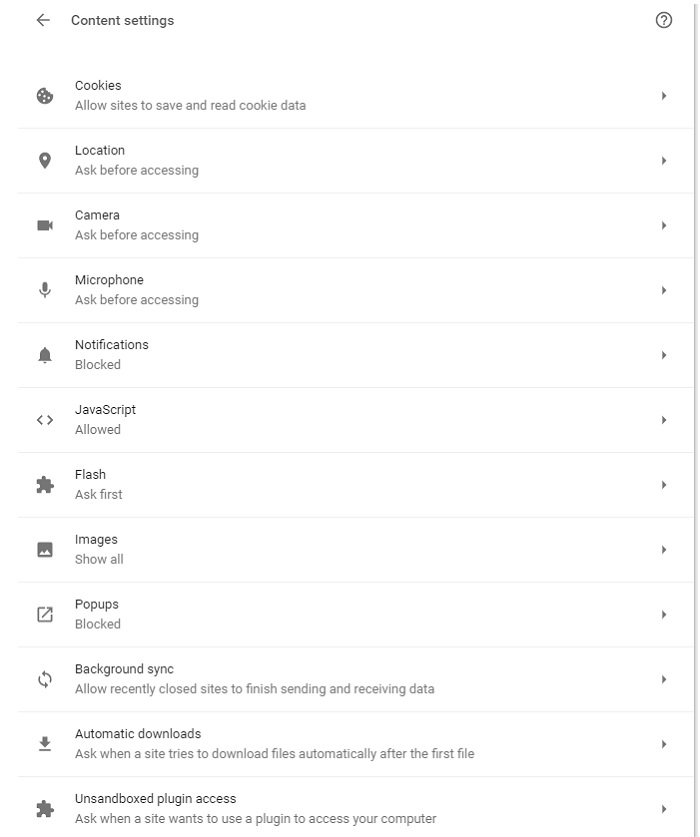The image showcases a settings screen from an application, predominantly featuring a white background. In the top left corner, there is a back arrow, followed by the text "Content settings" in the center, and a help icon on the far right. Below this header, there is a vertical list of items, each representing different configurable options within the application:

1. **Cookies**: Manage cookie settings.
2. **Location**: Control location access.
3. **Camera**: Manage camera permissions.
4. **Microphone**: Manage microphone permissions.
5. **Notifications**: Configure notification preferences.
6. **JavaScript**: Enable or disable JavaScript.
7. **Flash**: Manage Flash settings.
8. **Images**: Control whether images are shown.
9. **Pop-ups**: Currently set to blocked.
10. **Background Sync**: Option allowing recently closed sites to finish sending and receiving data.
11. **Automatic Downloads**: Requires a prompt when a site tries to download files automatically after the first file.
12. **Unsandboxed Plug-in Access**: Prompts when a site wants to use a plug-in to access your computer.

Each item is clearly listed to facilitate easy navigation and configuration of the application's settings.